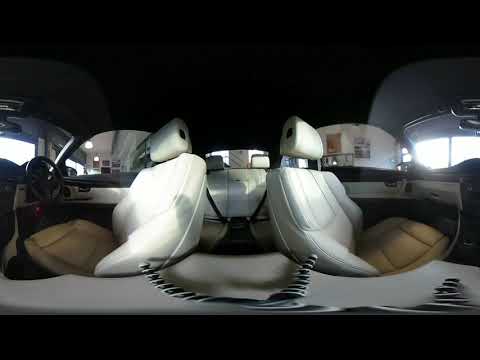This is a highly-detailed 360-degree photograph of the interior of a car, showcasing various elements within the vehicle. On the left side, there's the driver's seat, featuring a black steering wheel and white leather upholstery. Opposite the driver's seat on the right is the passenger seat, also upholstered in white leather. Due to the 360-degree nature of the photo, the seats appear to be tilted away from each other. Both front seats have adjustable white headrests, with the right one pulled up and the left one pushed down. 

The back seats are also visible, indicating it's a four-seat vehicle. The interior trim includes a mix of white and black elements; the lower half is predominantly white while the upper sections, including the roof, are black. A tripod stand, used to mount the 360-degree camera, is evident at the bottom center of the image.

Outside the windows of the car, it appears to be parked in a large garage or similar overhanging facility. The garage door is open, allowing daylight to illuminate parts of the vehicle's interior. Additionally, some pictures are hanging on the walls of the garage. The overall color scheme of the interior combines white and beige tones, with black being prominent in the steering wheel and upper trim.